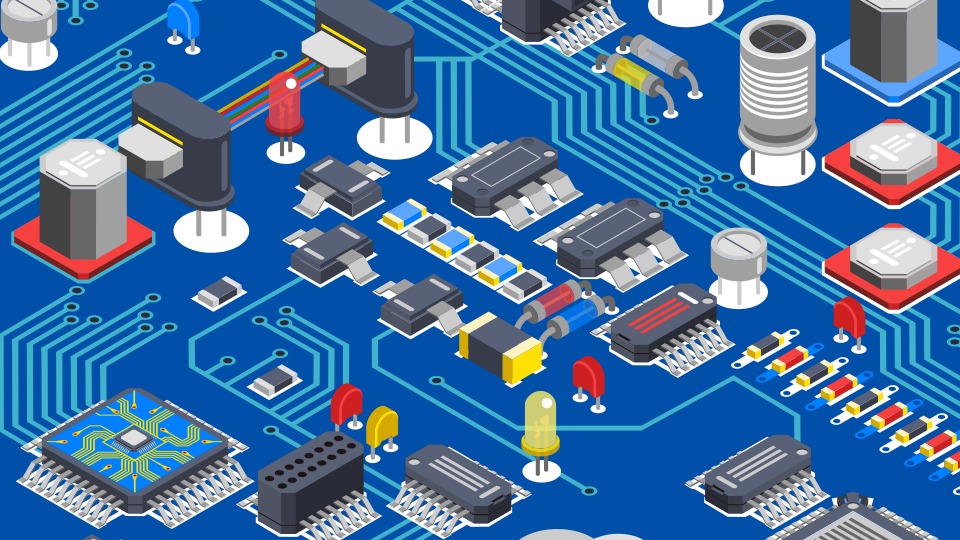The image appears to be a computer-generated visualization of an animated circuit board set against a rich, dark blue background. Intricate teal lines meander and zigzag across the surface, forming a web of connections between various electronic components. Each teal line terminates in a black circle, suggesting nodes or endpoints in the circuitry. The board features a diverse array of components in different geometric shapes, including squares, hexagons, tall cylinders, and rectangular prisms. Among these, some components stand out with vivid colors: silver elements resembling solar panels, yellow and red screws, and gray chips. Red squares with gray tops and red elements resembling popsicle tops with white circles underneath add further detail. This highly detailed depiction, reminiscent of a CAD drawing, intricately blends shades of blue, gray, red, and yellow, capturing the complexity and organized chaos of a circuit board.